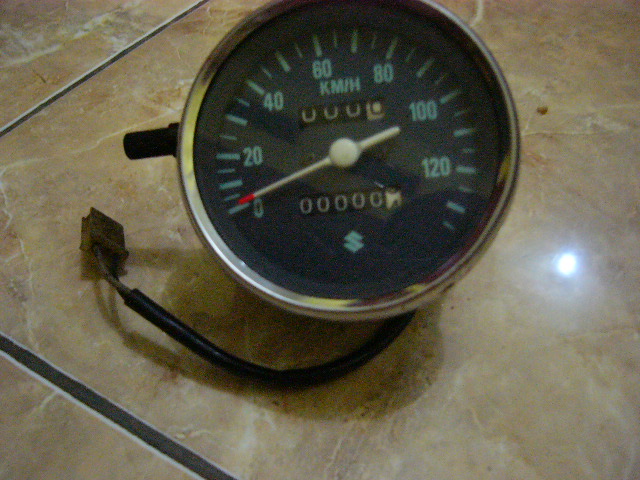The image depicts a motorcycle tachometer positioned on a marbled tile surface, likely a floor. The tiles are a light tan and cream color, interspersed with dark grout, creating a striking contrast. A flash of light reflects off the glossy tiles, enhancing the scene's detail. The tachometer is round, made of stainless steel, with a black dial featuring blue numerals. The numbers, marked in increments of 20, arc from left to right, ranging from 0 to 120. The odometer currently shows a mileage of 00000, with the last dial positioned between 3 and 4. A blue "S" possibly representing Suzuki is visible at the bottom of the tachometer. Above the tachometer numbers reads "KM/H", indicating the unit of measurement. A black cord, wrapped in electrical tape, extends from the tachometer, ending in a plug-in connector.